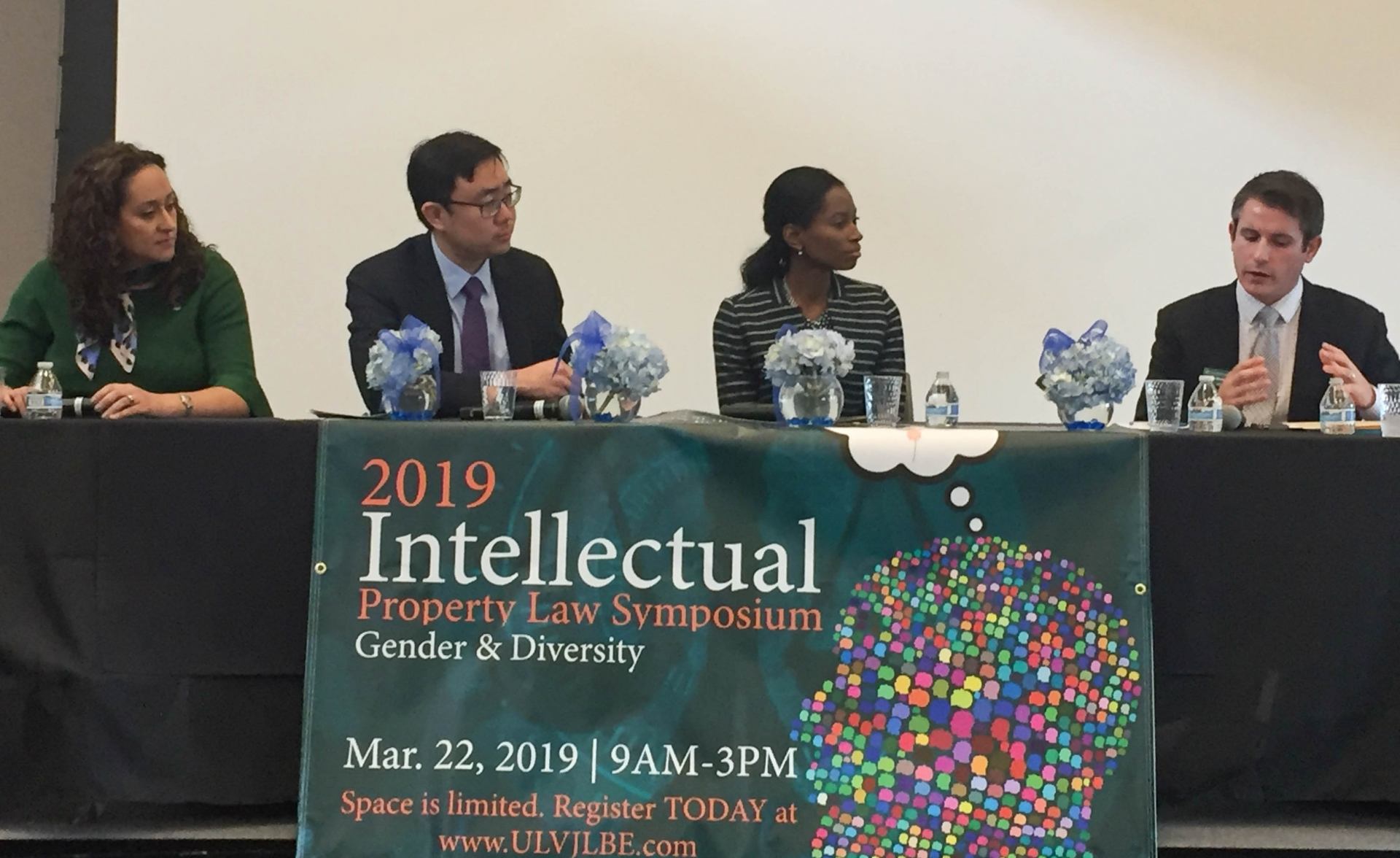The image depicts a 2019 Intellectual Property Law Symposium focused on Gender and Diversity, taking place on March 22nd, 2019, from 9 a.m. to 3 p.m. The scene is set at a conference where four diverse individuals are seated at a long table draped in a black tablecloth on a stage. The table features clear glass vases filled with white and blue flowers, and glasses of water are placed in front of each speaker.

On the front of the table hangs a large green banner adorned with an artistic depiction of a human head composed of multi-colored dots, primarily in green, blue, and purple. To the left of this graphic, white and red text reads: "2019 Intellectual Property Law Symposium, Gender and Diversity, March 22nd, 2019, 9 a.m. to 3 p.m. Space is limited, register today."

Seated from left to right are:
1. A woman with long brown hair wearing a green long-sleeve blouse with a scarf tied around her neck.
2. An Asian man with dark hair, glasses, a blue button-up shirt, and a dark blue tie.
3. A Black woman in a black and white striped dress.
4. A white man, currently speaking and gesticulating, with dark hair parted to the side, wearing a button-up white shirt, gray tie, and suit jacket.

Behind them is a large projection screen, although it is not in use at the moment. The atmosphere suggests a formal and informative gathering with an emphasis on intellectual property law, gender, and diversity themes.